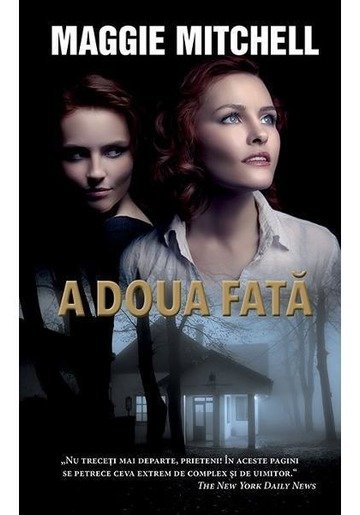This image, likely the front cover of either a book or a movie advertisement, features various elements with notable text placements and distinct aesthetics. Dominating the top portion is the author's name, "Maggie Mitchell," followed by the title, "Adua Fata," positioned centrally. The bottom section contains a description in a foreign language. The primary visuals include two women: one with reddish-brown hair glancing slightly to the side with a somewhat sinister expression, and the other, dressed in a white blouse, looking upwards as if gazing at something unseen. The women are depicted against a dark, black background. Below them is an eerie, fog-shrouded scene showing a white house at night, surrounded by tree trunks. The palette includes hues of black, white, brown, off-red, pink, yellow, and gray, contributing to an atmospheric and slightly mysterious ambiance.